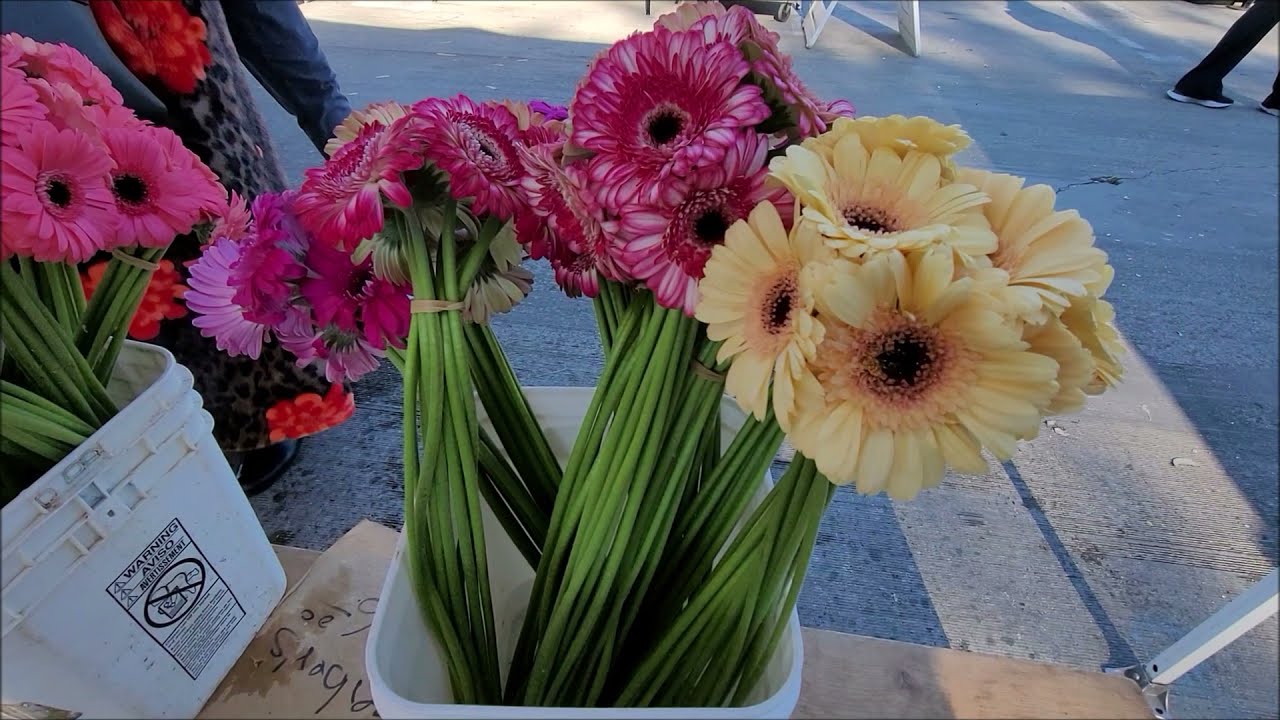In this detailed outdoor scene, a vibrant array of flowers is displayed in plastic buckets against the backdrop of a bustling environment, likely a farmer's market evident from the people walking through and sandwich boards for advertising. Two white plastic buckets are centrally positioned at the bottom of the image; the one in the middle is filled with bundles of flowers, featuring several bunches of red flowers on the left and a single bunch of yellow flowers on the right, all with long green stalks and many small petals. The bucket on the bottom left corner contains red flowers of the same type. Pedestrians, including a pair of black tennis shoes and black and white sneakers, pass by on the cement ground. A woman wearing a leopard print vest is visible near the flowers, and to the left, partially obscured, stands a person in a brown jacket with a red scarf. In the background, the pavement of the street further emphasizes the lively setting.